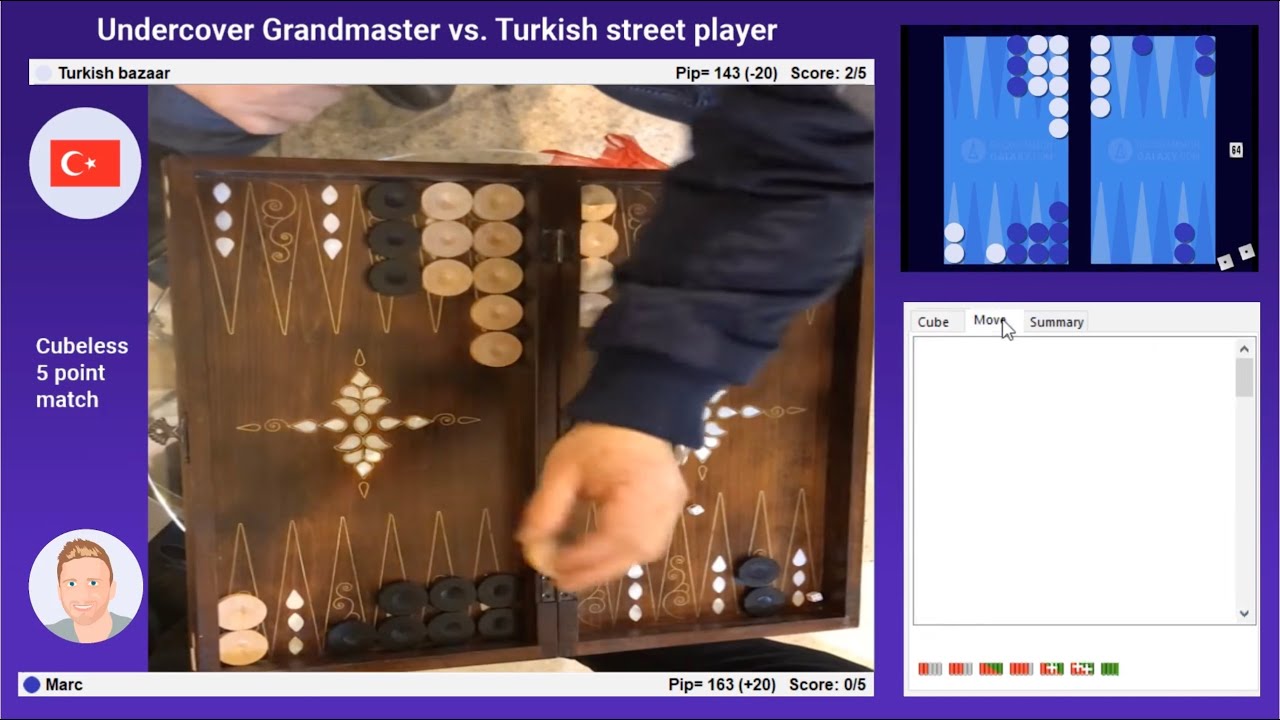The image displays a detailed digital screen capturing a gripping match titled "Undercover Grandmaster vs. Turkish Street Player," inscribed in prominent white letters against a bluish border at the top. The backdrop includes a gray bar labeled "Turkish Bazaar." Central to the image is a close-up of a wooden backgammon board characterized by its dark brown hue and intricate triangular patterns. The board is equipped with black and white chips arranged for gameplay. Visible on the board's left side is an arm clad in a black jacket, poised to move a piece.

On the left side of the screen, a blue circle features the Chinese flag, while adjacent text states "cubeless five-point match." Further details include another blue circle depicting a cartoon man with yellow hair, blue eyes, and labeled "Mark" below. A notable red circle with a crescent moon and star—symbolizing the Turkish flag—also appears on the left side. On the right side of the screen, a dark square holds an animated rendition of the backgammon game with blue and white geometric designs. At the bottom right, a white square contains additional text.

This elaborate scene captures the intensity and international flavor of the game, with a player’s arm actively engaging with the backgammon board, suggesting a moment of strategic gameplay.